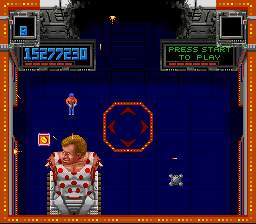A screenshot from a retro 1980s-style video game displays a vivid scene. The border of the image is predominantly red, adorned with an array of orange, yellow, and green square patterns that frame the screen, leaving the top center part with a clear ruby hue. Within this retro-styled border, a central area features a scene laden with nostalgic pixel art.

The background consists of a blue-tiled floor with both rectangular and square tiles meticulously arranged, giving the sense of a classic game environment. Amidst this setting, a large animated character reminiscent of Richard Simmons lies on a white medical table. This character sports red-and-white leotards and has reddish-brown hair, but notably lacks visible arms or legs, adding a quirky charm to the depiction.

Adding to the animation, black smoke and white rectangular blocks appear near the top central portion of the screen, contributing to the game's distinctive atmosphere. In the upper right-hand corner, bold green text instructs viewers to "Press Start to Play." Additionally, another game figure stands nearby, characterized by a red shirt, blue pants, perhaps gray or white gloves, and a blue hat, enhancing the nostalgic allure of this retro game scene.